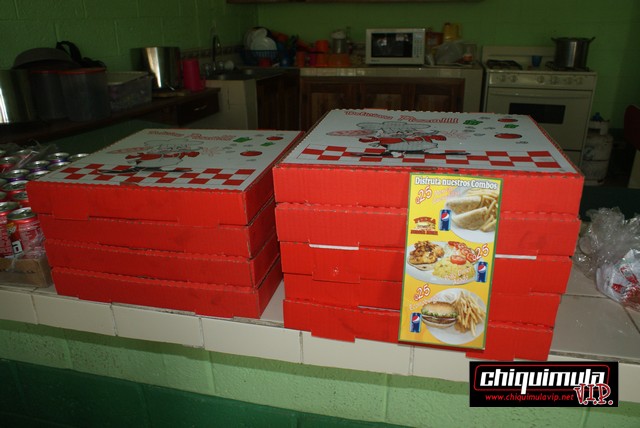The photograph features two stacks of pizza boxes on a green and white tiled countertop within a kitchen setting. The boxes are predominantly red with white tops that feature a checkered design and an image of a character. The stack on the left comprises four boxes, while the right stack has five. The counter also holds a box containing aluminum soda cans. The kitchen background shows a stove on the right, a microwave on the left counter, and a green wall. Additionally, a black bar with white text reading "CHIQUIMULA" and some red text, which is difficult to read, appears in the lower right corner of the image. There's also a yellow pizza menu hanging off the right stack of boxes.